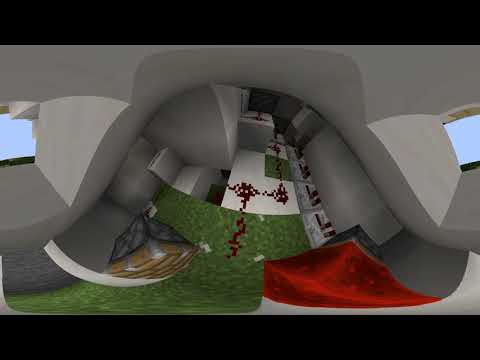A digitally created image showcases a bird’s-eye view of an enclosed room rendered in a video game, possibly Minecraft or a computer graphics scene. The perspective is slightly distorted, resembling a fisheye lens effect. The room has gray concrete-like walls, punctuated by windows on both the left and right sides, revealing a simulated blue sky. The flooring features a mix of green carpeting and a red carpet, alongside a checkerboard pattern of green and white. Central to the image, a black table is flanked by a gray chair on the left and a gray couch on the right. A brown, squiggly, line-based trail, composed of squares, runs across the scene. The coloration varies, predominantly featuring gray, white, green, red, and brown tones, creating a visually complex and somewhat random composition. A black border surrounds the entire image, contributing to the impression that it is a screenshot captured from a digital platform.